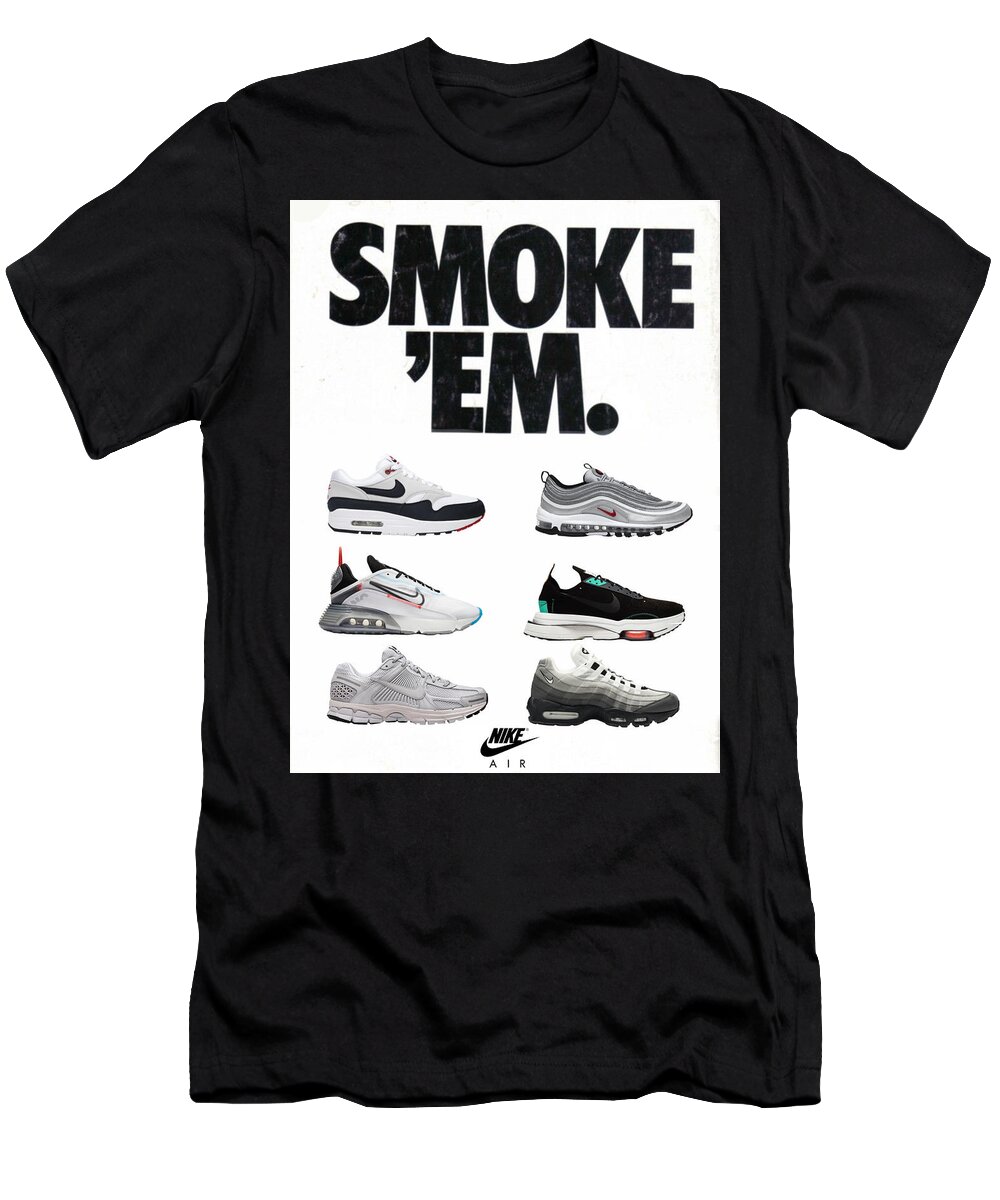This product image features a black, short-sleeved, crew-neck Nike Air t-shirt. The t-shirt is adorned with a prominent white rectangle occupying the entire front. Within the upper third of this rectangle, bold black uppercase lettering spells out "Smoke 'Em." Below this text, there are images of six different Nike sneakers arranged in three rows and two columns. The specifics of the shoes are as follows: the top left pair is white with a black Nike swoosh and an air cushion sole; the top right pair is gray with a small red Nike swoosh and enhanced tread, resembling running shoes; the middle left pair is white with orange accents; the middle right pair is black with aqua highlights and a sock-like design; the bottom left pair is entirely white, reminiscent of a "dad" sneaker; and the bottom right pair transitions from black soles to white laces in an ombre effect. Centered at the bottom of the rectangle, in a smaller font, is the Nike Air logo, featuring the word 'Nike' within the swoosh above the word 'Air.'